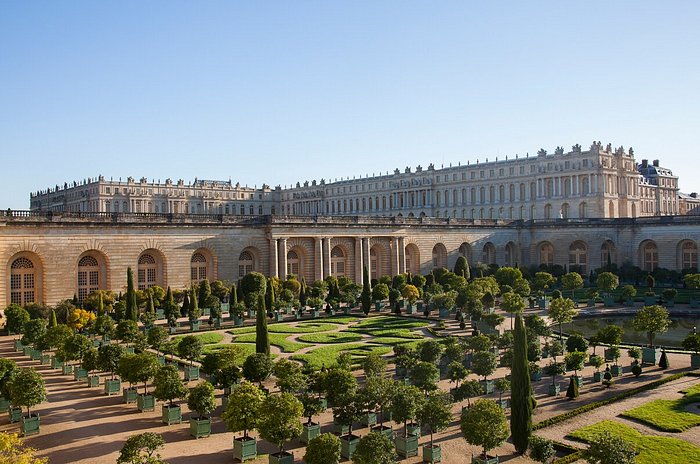The image showcases the partial angled view of a meticulously maintained castle garden. The manicured gardens feature decorative, maze-like grass installations adorned with precisely trimmed topiary trees and boxed plants neatly lined along light brown pathways, which may be made of cement or dirt. Within the garden, circular and slender, tall trees are artfully arranged. The background reveals a stone structure constructed from light, sandy-colored bricks, featuring a series of rounded arched windows and four sets of columns. Above this structure, the L-shaped castle extends, with its taller section wrapping around the stone building. The sky overhead is a vivid, cloudless blue, enhancing the grandeur and fairy tale-like quality of the scene, reminiscent of a royal castle straight out of Alice in Wonderland.